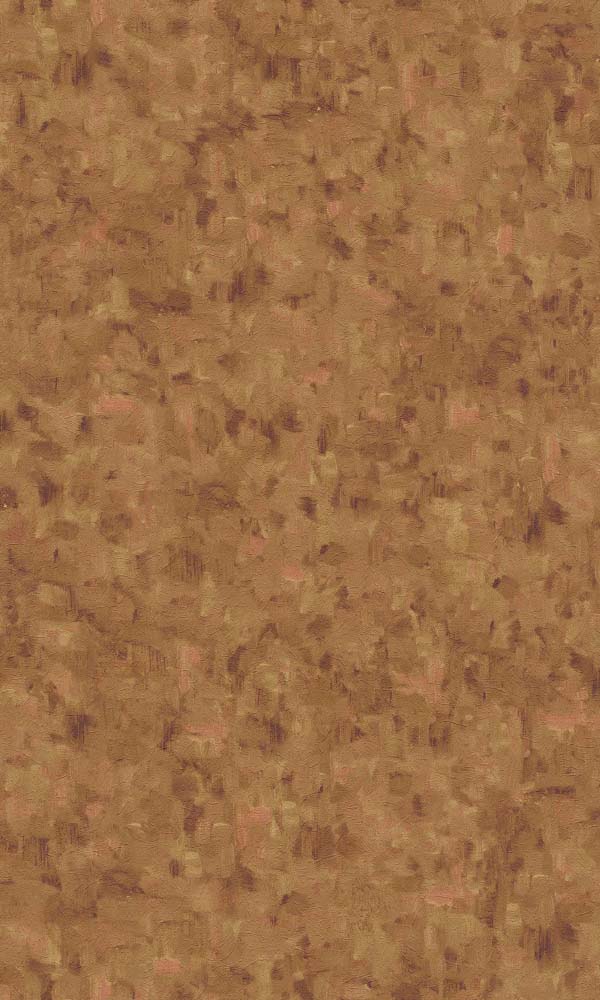The image depicts a long rectangular canvas that resembles a textured, multicolored cork surface. It has an overall camel or brownish-orange background with various blotches and swatches of color, including shades of dark brown, chestnut, tan, beige, and light pink salmon. The colors are inter-blended and presented in a way that makes the surface appear almost like marble or granite. The brush strokes are randomly placed, creating a non-uniform, organic pattern. From a distance, the image appears as a dirty brown expanse, but upon closer inspection, the individual shades and textures become evident. It evokes a sense of looking at a bulletin board in a break room or school hallway, capturing a mundane yet intricate surface detailed enough to be used as an iPhone wallpaper.